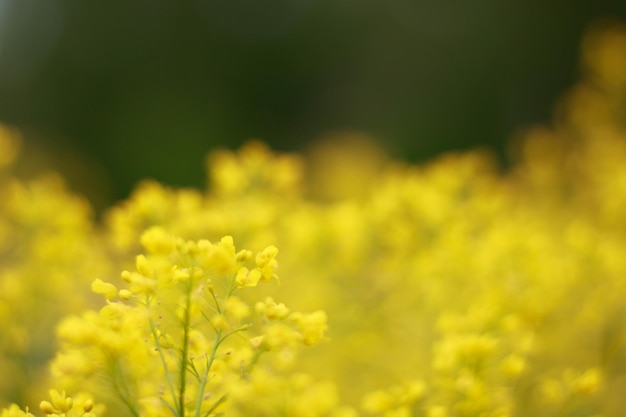This outdoor photograph captures a vibrant field of wild yellow flowers. The focal point of the image is a cluster of tiny yellow flowers, reminiscent of buttercups, perched on slender green stems. This primary bunch, positioned slightly off-center to the left, comprises three shoots adorned with closely grouped blooms, and stands out sharply against the blurred background. The backdrop reveals an expansive array of similar flower clusters, progressively becoming more out of focus into a haze of yellow and green. This creates a dreamy scene where the detailed foreground contrasts with the vast, indistinct expanse of flowers extending into the distance.